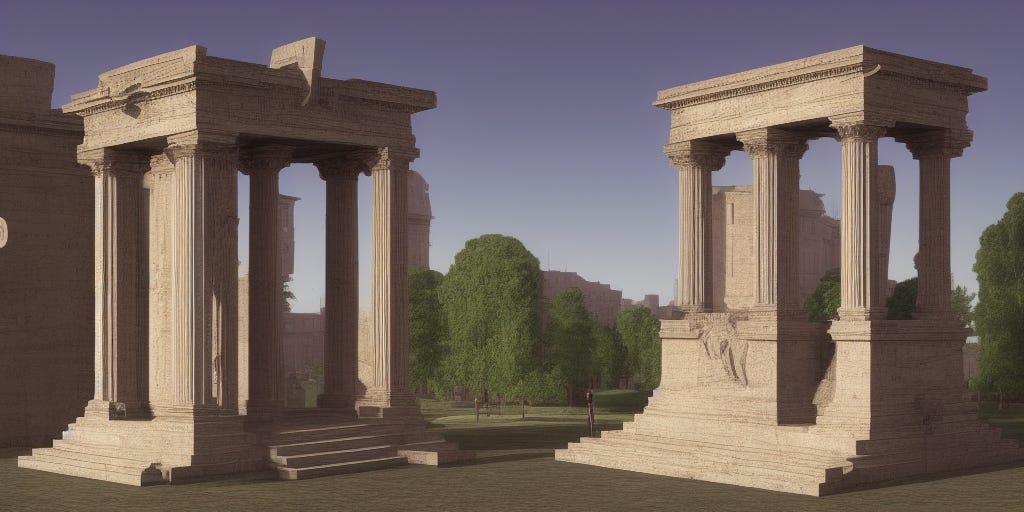The image appears to be a detailed drawing of two freestanding structures modeled in the classical Greek architectural style. Each structure features large stone marble-like columns and steps leading up to an interior section. Both structures are rectangular and face towards one another at the center of the composition. The columns, consistent in height, support the buildings' tops, and you can see through to the opposite side, suggesting an open design.

Surrounding the structures, the background reveals tall, green bushy plants and trees half the height of the buildings, indicating a lush environment. In the distance, there are indistinct and grayed-out structures, perhaps additional buildings or high rises, creating an impression of urban surroundings. The sky above has a dark blue hue, adding depth to the scene.

The ground in the foreground appears solid white, which might be marble or a different type of stony material, contributing to the ancient Greek ambiance. Additional elements include the understanding that the land does not resemble an ancient Greek locale but more of a contemporary park or playground setting.

Overall, while the image does capture the essence of ancient Greek architecture, the surrounding elements suggest it might be a modern recreation in a more current environment, perhaps an illustration rather than a photograph.